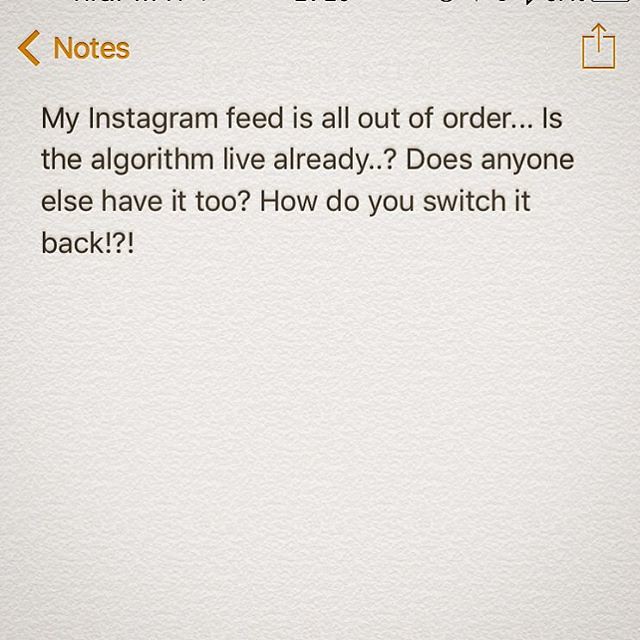The image is a square screenshot of an iPhone's Notes app with a beige background. In the upper left corner, there's an orange arrow icon next to the word "Notes," which allows navigation back. The upper right corner features an orange upload icon, indicative of sharing options. The main content of the screenshot is positioned towards the top in black text, reading: "My Instagram feed is all out of order. Is the algorithm live already? Does anyone else have it too? How do you switch it back?!" The lower portion of the image remains blank, highlighting the simplicity of the Notes app interface.